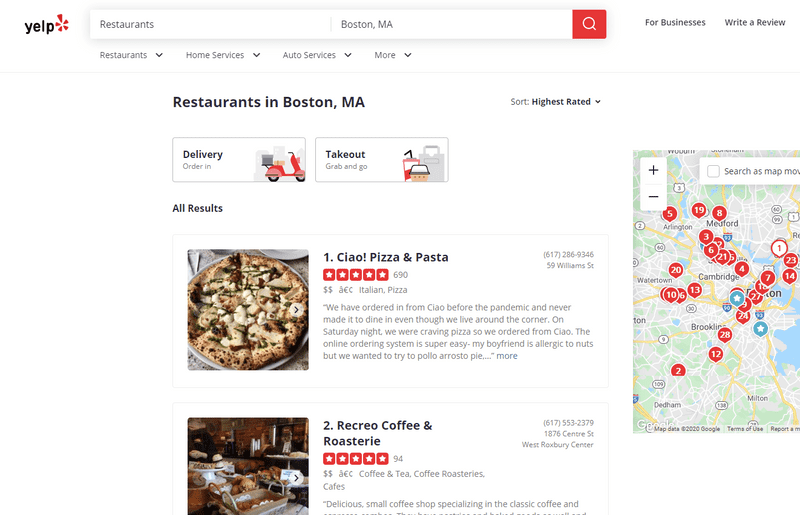This is a detailed screenshot of a Yelp page highlighting restaurants in Boston, Massachusetts. In the upper right-hand corner, the iconic Yelp logo is visible. The page features a clean white background with black text, and the star ratings are prominently displayed in red. A navigation menu with drop-down options for categories like Restaurants, Home Services, Auto Services, and more is situated at the top. The 'Restaurants' category is selected, specifically focusing on Boston, Massachusetts, as indicated by the heading "Restaurants in Boston, Massachusetts."

Below the heading, there are two prominent rectangular buttons labeled 'Delivery' and 'Takeout,' followed by a sorting option that defaults to 'Highest Rated.' The results section is listed as 'All Results,' but only two establishments are visible in the screenshot.

The first result is "Chow Pizza and Pasta," boasting an impressive five-star rating. To its left, there is a photograph showcasing a white pizza adorned with mushrooms, hinting at the restaurant’s delectable offerings. The second result features "Recreo Coffee & Roastery," also holding a perfect five-star rating. Accompanying this listing is a thumbnail image providing a glimpse into the cozy interior of the café.

To the right of the listings, a sidebar map marks the locations of the showcased restaurants, providing a convenient visual reference for potential visitors.